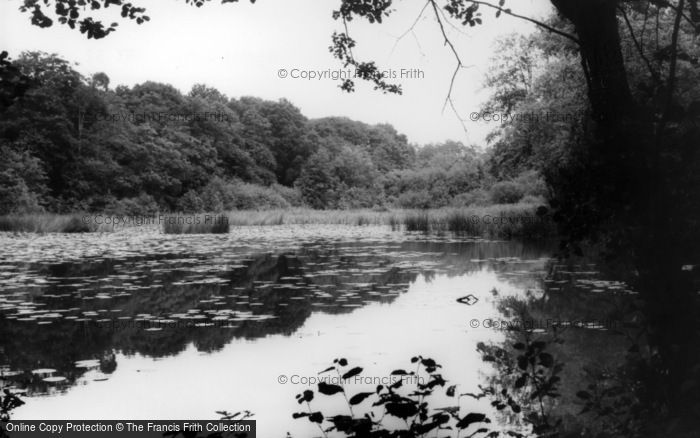A black and white photograph captures a serene lakeside landscape. The tranquil scene features a small, still lake framed by a mix of lush vegetation including ferns, tall grasses, and bushes with large teardrop-shaped leaves on the bottom right. Trees and various plants reflect off the water’s surface, contributing to the peaceful ambiance. The foreground displays detailed outlines of flora while the background reveals taller trees as the eye moves further into the distance. The sky is white, contrasting with the various shades of gray that dominate the scene. Overlays of semi-transparent gray and solid white text appear on the image, reading "copyright Francis Frith" at the top center and "online copy protection, copyright the Francis Frith Collection" at the bottom left. The scene suggests an untouched, natural environment, reminiscent of a swampy area or a secluded pond.